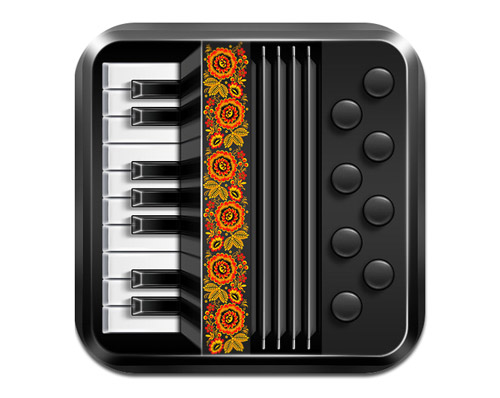The image features a highly detailed, computer-generated depiction of a miniature piano-like keyboard, centrally positioned on a solid white background. The object is a sleek, shiny black square with rounded edges, suggesting it could be made of either metallic material or plastic. The left side showcases a set of piano keys, containing 10 white keys and seven black keys arranged in the pattern of two black keys, followed by three black keys, and finishing with two more black keys atop the white keys.

Dominating the central portion of the object is a narrow vertical strip embellished with a floral pattern. This colorful design features six vertically aligned flowers with reddish-orange petals and orangish-green leaves extending from each blossom. 

To the right of the floral strip, a vertical louvered opening stretches from top to bottom, likely functioning as a speaker grill. The far right side of the object is adorned with eight round black buttons arranged in a zigzag pattern. The top left and right corners of the object reflect light, indicating a light source from above, contributing to the overall shiny appearance of the piano-like keyboard. There is no text present in the image, which displays colors such as black, white, red, orange, gray, yellow, and green. The composition suggests that the object could be part of a musical setting, a classroom, or an online sales listing.